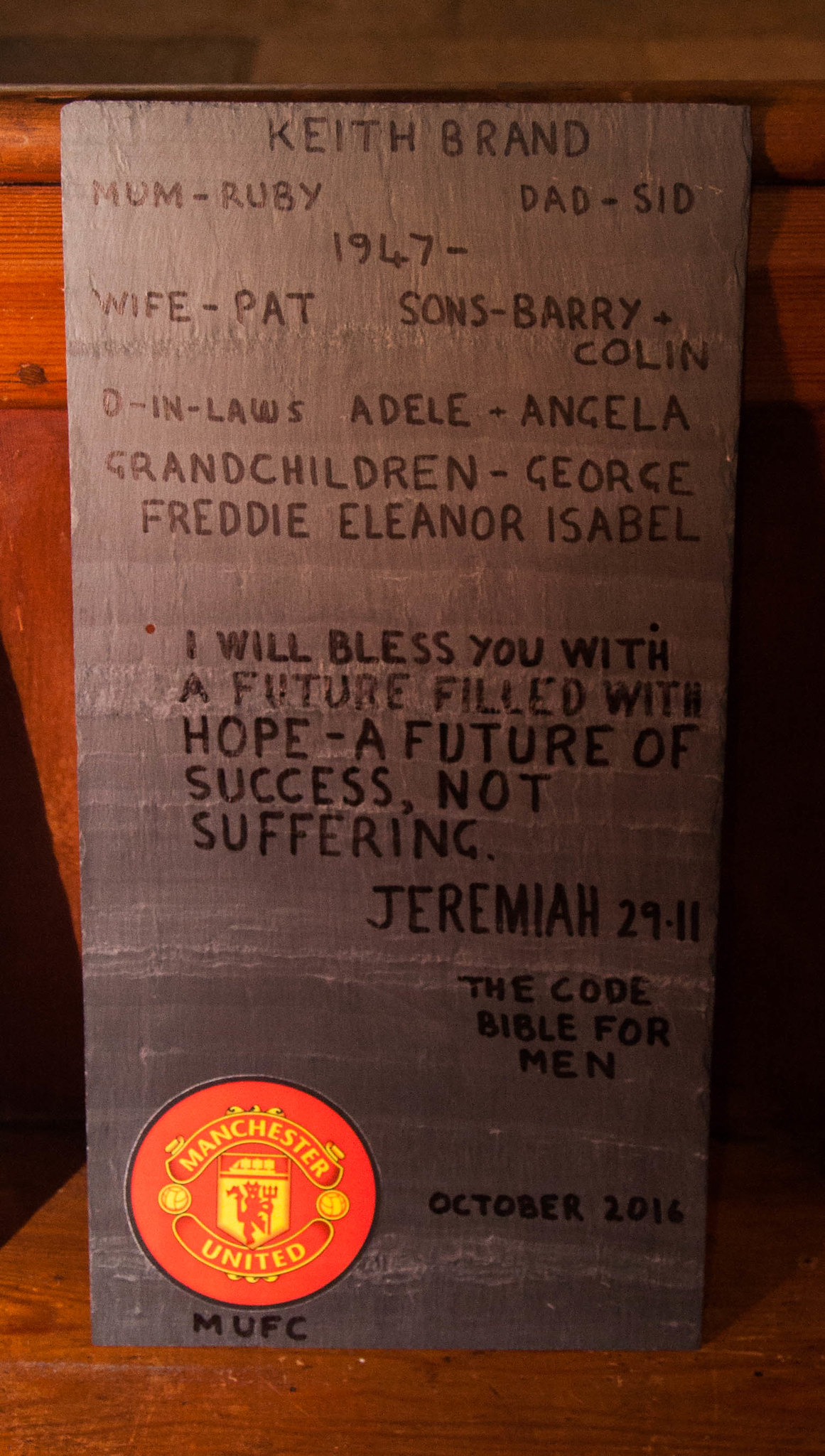The image depicts what appears to be a detailed and possibly hand-drawn memorial or tombstone honoring Keith Brand. At the top of the display is the name "Keith Brand." The inscriptions list several family members, including his mother Ruby, father Sid, and wife Pat, along with his sons Barry and Colin. Extended family members include daughters-in-law Adele and Angela, and grandchildren George, Freddie, Eleanor, and Isabel. The inscription also features a Bible verse from Jeremiah 29:11: "I will bless you with a future filled with hope, a future of success, not suffering." Below the biblical quote, a reference to "The Code Bible for Men" is noted, followed by the date October 2016, which might indicate the time of Keith Brand's passing. The stone is brownish with dark brown or black writing. At the bottom left corner sits the Manchester United Football Club logo—red and yellow in color, within a circular emblem, accompanied by the acronym "MUFC." The background appears to be supported by a wooden structure, enhancing the prominence of the memorial stone in the foreground.